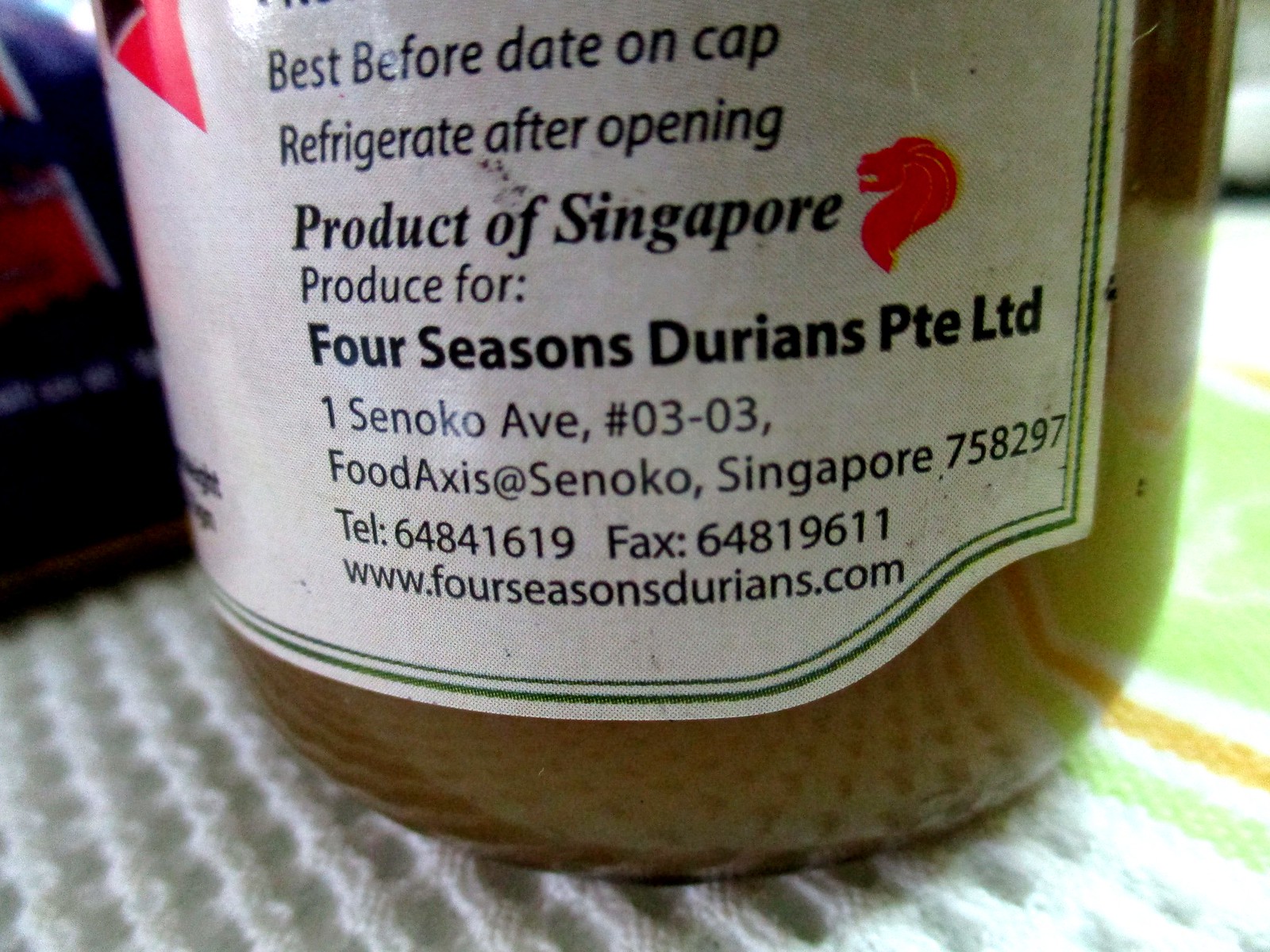The image features a close-up view of a jar that appears to contain a brown substance, possibly a condiment or spread. The jar is labeled as a product of Singapore and is produced for Four Seasons Durians, PTE LTD, located at 1 Senko Avenue, #03-03 Food Access at Senko, Singapore, 758297. The label is predominantly white with two green stripes at the bottom, and also features a red and black emblem on the front. A small stylized lion head icon is situated next to the word "Singapore." It is noted that the writing on the label is in black, with specific instructions to refrigerate the product after opening and to check the best before date on the cap. Contact information including a phone number (64841619), a fax number (64819611), and a web address (www.fourseasonsdurians.com) is also provided. The jar is placed on a white placemat, and sunlight shines from the right, illuminating the setup.